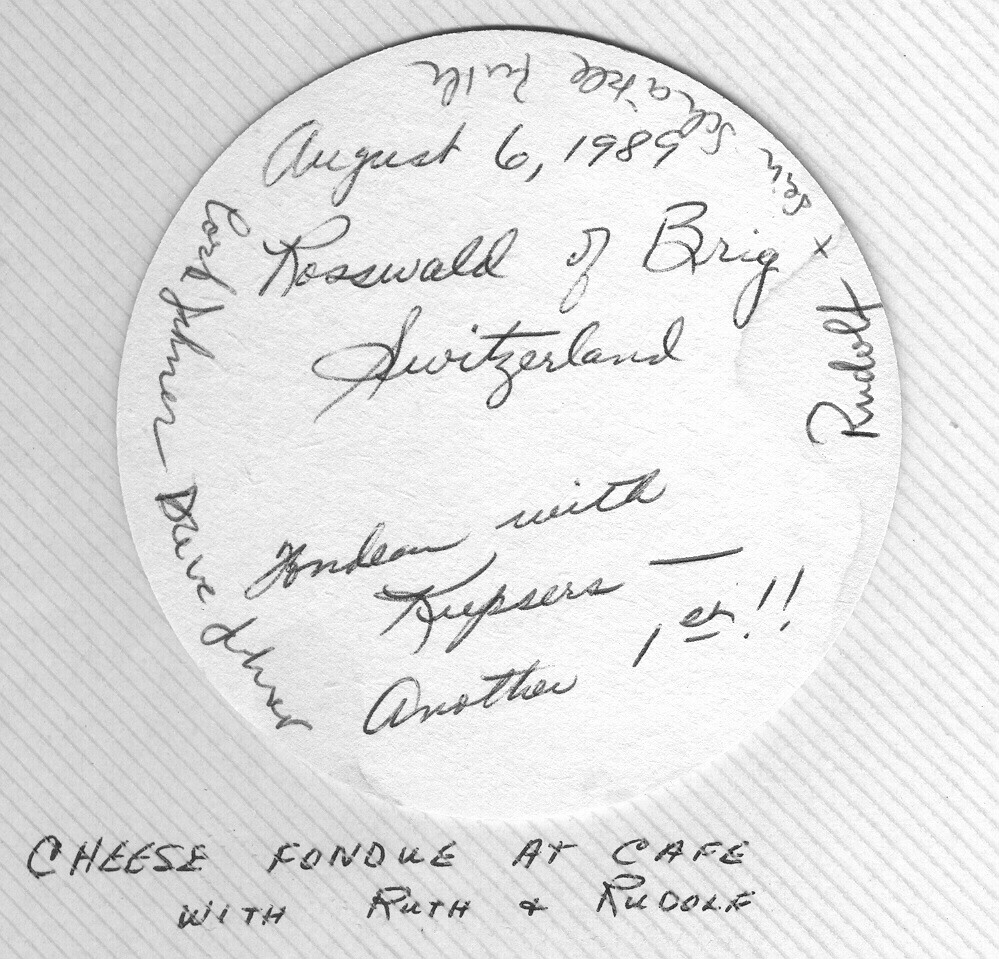The image depicts a white circular label adorned with tight, cursive handwriting. The label appears to be placed on a lined, possibly striped, background which has light blue diagonal stripes. The top of the label features the date "August 6, 1989." Below that, the text reads "Rosswald of Brigg, Switzerland," followed by other text that mentions a memorable event. The bottom of the label states in cursive, "Cheese fondue at cafe with Ruth and Rudolph." Additionally, the border of the label is closely inscribed with more cursive text that includes the name "Rudolph." The scene is on a tabletop, where the label stands out against the brighter right side, which is illuminated compared to the slightly darker left side of the background.